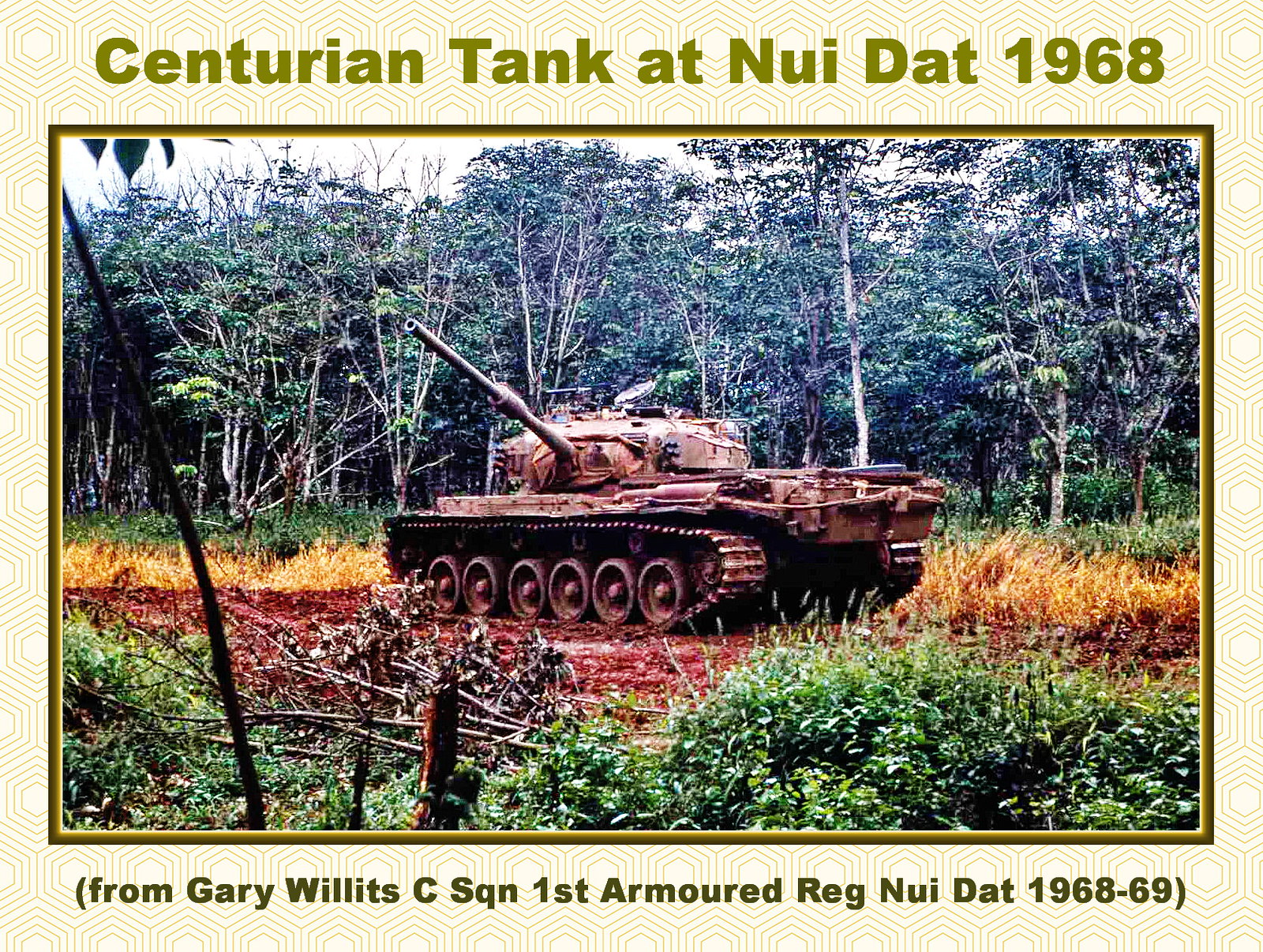This photograph, resembling a vintage postcard, showcases a Centurion Tank situated at Nui Dat in 1968, a pivotal vehicle from the Vietnam War. The image captures the right side of the tank, revealing its robust design with distinctive treads wrapped around six wheels on each side, and its turret slightly turned to the left. The tank, painted in a camouflaged brownish-green hue, rests on a dirt path seemingly forged by the passage of military equipment. Surrounding the scene is a mix of green, yellow, and brown grass and shrubs, with dense, tall, bushy trees forming the backdrop. A hint of the sky peeks through the canopy. The border of the photo features green text above and below, stating, "Centurion Tank at Nui Dat, 1968" at the top, and "From Gary Willett's C-Squadron First Armored Regiment, Nui Dat 1968-69" at the bottom, marking it as a historical relic from a soldier's collection.